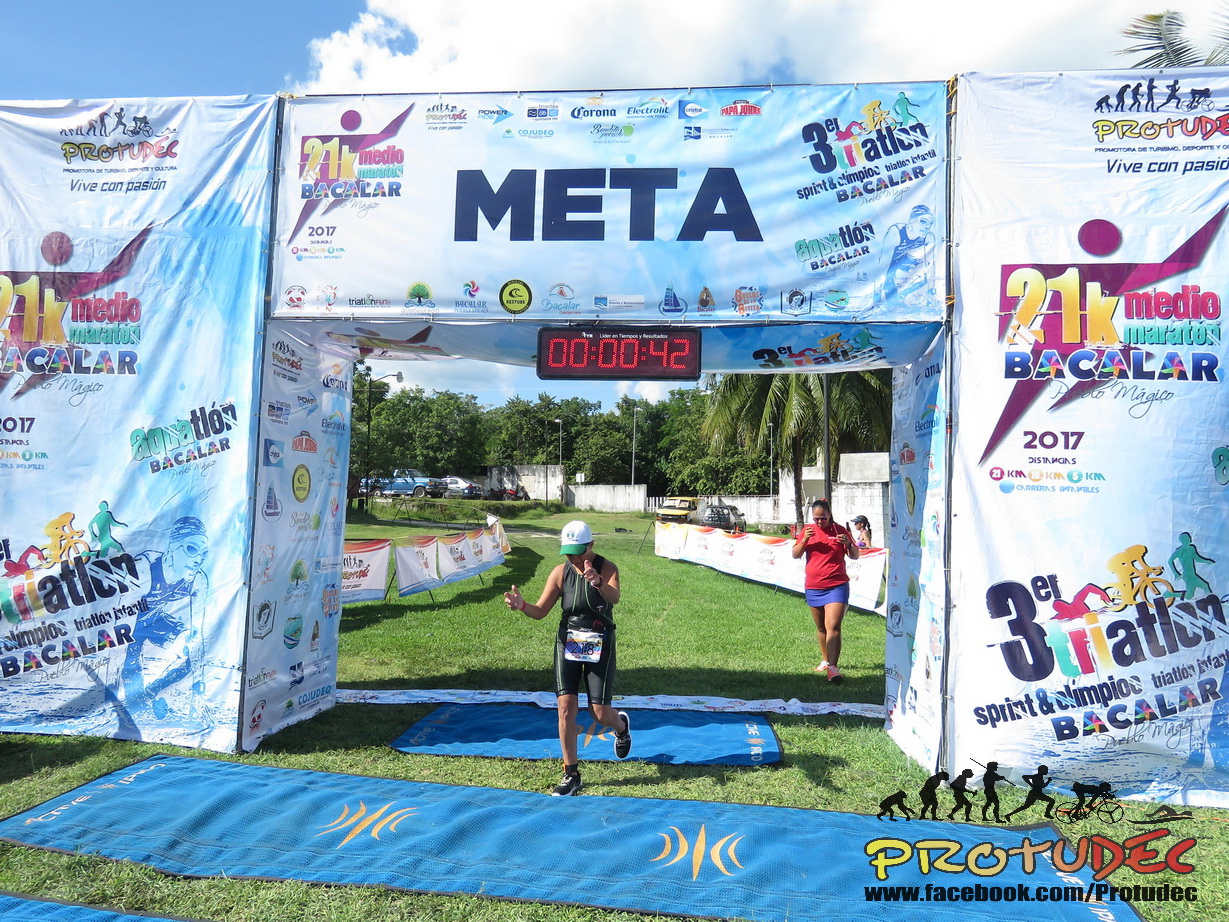In this vibrant photo of a triathlon event, a woman is captured triumphantly crossing the finish line. With her arms raised in victory or giving thumbs up, she sports a white and green hat, black athletic wear, and black tennis shoes. Her runner's bib prominently displays the number 2118. The finish line area features blue mats on the ground and is adorned with a large tunnel-like structure made from poles and tarps, covered in advertisements and event names such as "Rear Triathlon Sprint" and "Olympiak Bakalar," as well as various sponsors like Corona, Papa Jones, and others.

A second woman, dressed in a red shirt, blue skort, and tennis shoes, is diagonally behind the first, just about to cross into the finish line area. She wears sunglasses but doesn't appear to be a participant. The scene is set against a backdrop of green grass, palm trees, and other distant trees, with a parking lot holding several cars, including a blue truck and a silver car. A van, parked just beyond the fencing made of advertising tarps, stands to the right.

The sunny day with clear blue skies and thick white clouds adds to the celebratory atmosphere, with the sunlight streaming from the center-left of the image. A digital timer above the finish line displays 00:00:42, indicating the time elapsed in this segment of the race. In the bottom right corner, a logo showing the evolution from a monkey to a person running, biking, and swimming is visible, alongside the text "www.facebook.com/prototech."